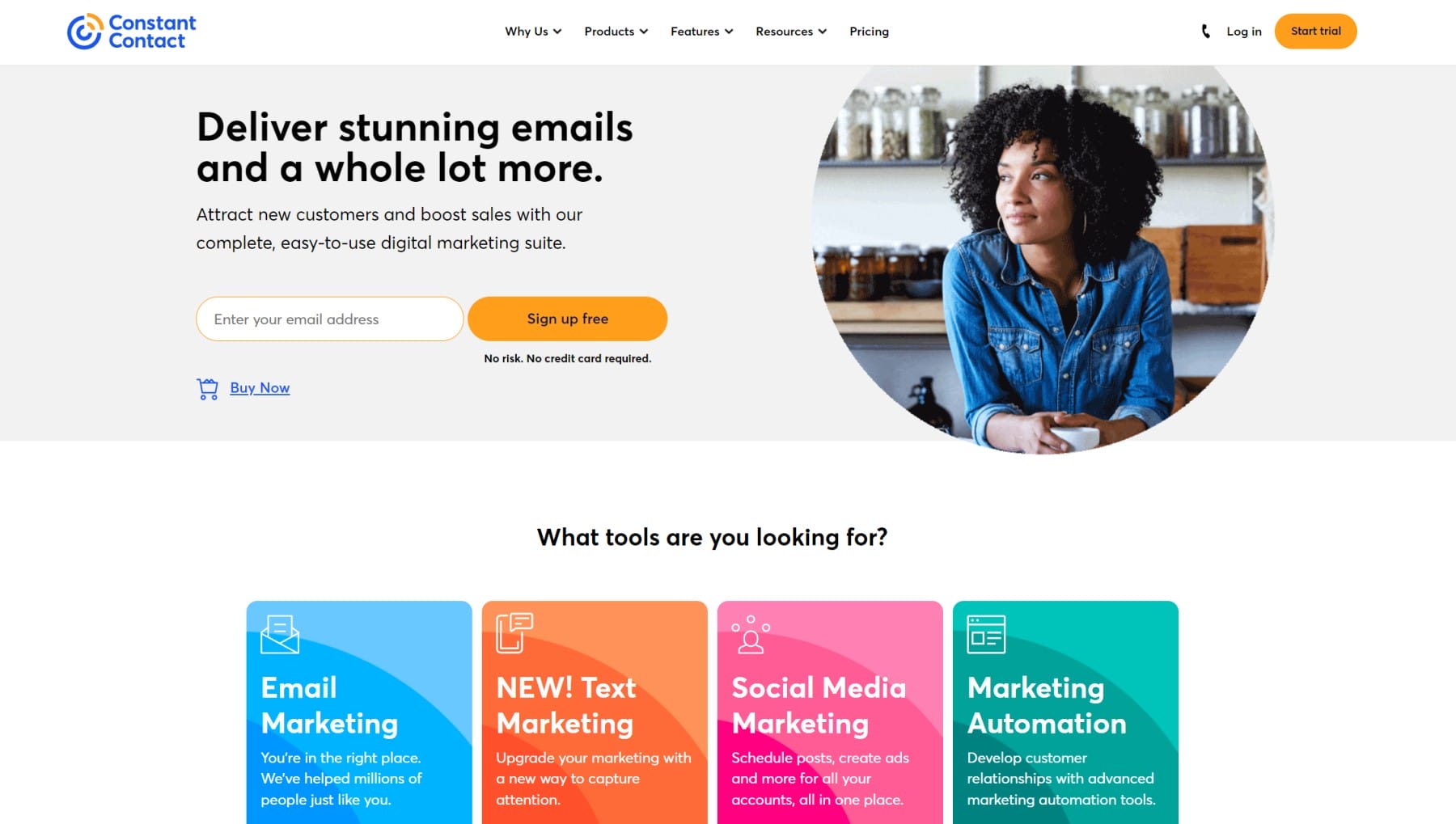This is a cropped screenshot of a Constant Contact desktop web page. At the top left corner, the Constant Contact logo is prominently displayed, with the text in a bold blue color. Centered across the top of the page are several categories: "YS," "Products," "Features," "Resources," and "Pricing." To the far right, there is a telephone icon, a "Login" text link, and an orange button labeled "Start Trial."

Below the navigation bar, a large gray rectangular box dominates the screen. On the left side of this box, a bold black headline reads "Deliver Stunning Emails and a Whole Lot More." Directly beneath this headline, smaller black text states, "Attract New Customers and Boost Sales with our Complete, Easy-to-Use Digital Marketing Suite."

Centered under this text is a search bar with the placeholder text "Enter Your Email Address" in small gray font, accompanied by an orange "Sign Up Free" button in small black font to its right. Beneath the search bar and to the left, there is a blue "Buy Now" hyperlink with a shopping cart icon adjacent to it.

At the bottom of the screenshot, a bold black headline asks, "What Tools Are You Looking For?" Immediately below this question are four colored square boxes each representing different tools: "Email Marketing" in blue, "Text Marketing" in orange, "Social Media Marketing" in pink, and "Marketing Automation" in bluish-green.